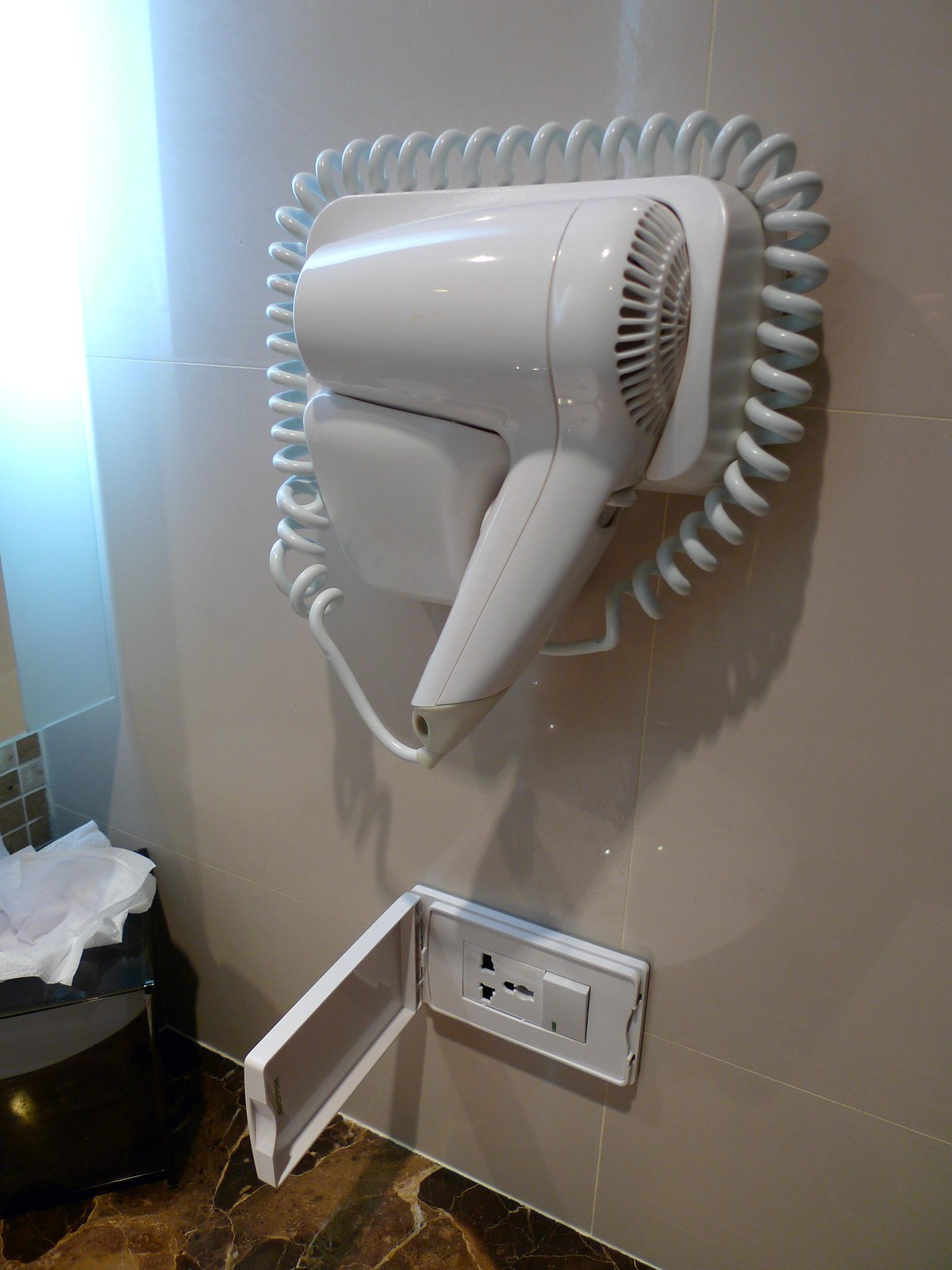The image depicts a small, white hairdryer mounted on a tan-tiled wall in a bathroom, possibly within a hotel room. The hairdryer features an old-fashioned coiled cord wrapped around it. Directly below the mount is a covered plug, which appears to be a European-style outlet with the cover open. The bathroom wall also has a mirror accompanied by smaller tiles underneath it. Below the mirror, there's a light tan and dark brown marbleized counter, upon which sits a brown tissue box. To the left side of the image, there is some white paper or tissue on a darker surface, possibly hinting at the presence of a black bag or an object on the counter, and a bright light suggests a nearby window.